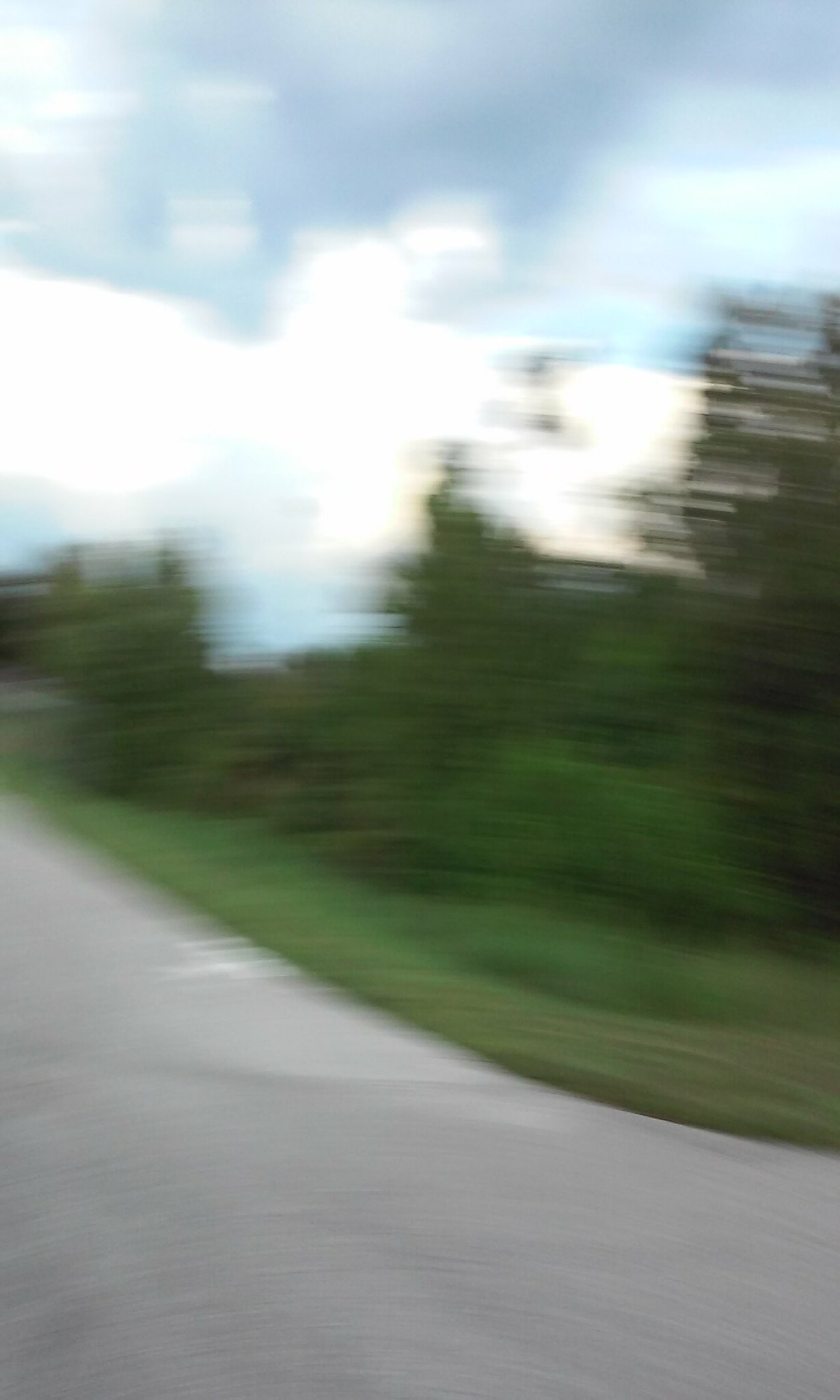This vertical, color photo captures a blurry image of a roadway in a rural area, possibly taken from a moving vehicle or by someone running at full speed, resulting in distorted visuals. The road, made of gray concrete or asphalt, occupies the left side of the image, though it's difficult to discern any markings due to the blur. On the right side, there's a treeline with green grass and possibly bushes in the mid-ground. The background features a blue sky interspersed with white clouds, all rendered with a pronounced blur that suggests motion. The overall effect is a hazy and dynamic representation of a sunlit day in a quiet, natural setting.